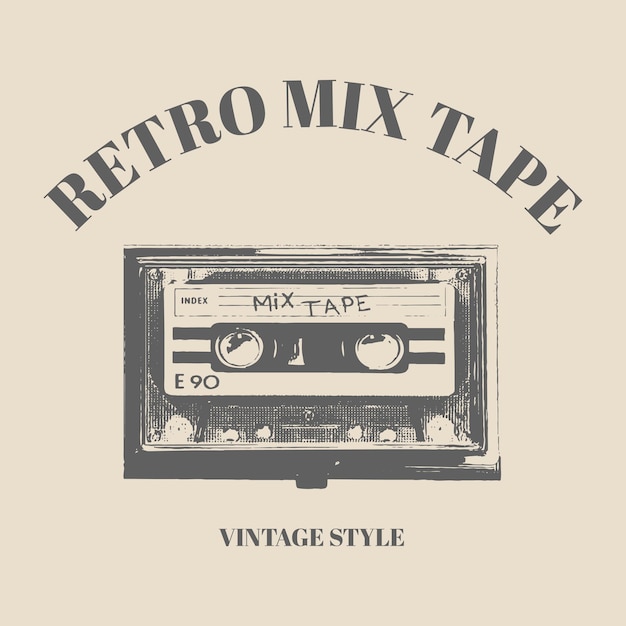The image is a promotional graphic or t-shirt design featuring a squared layout with a light gray to tan background. At the top, there is large black text curving upwards that reads "Retro Mix Tape." Below this text, a drawing of an old-fashioned cassette tape with a checkered black edge appears. The cassette tape is depicted with a white label area displaying the words "Mix Tape" and the usual space for writing an index. On the left side of the cassette's label, it reads "E90." Beneath the cassette tape, more black text states "Vintage Style." The entire image has a faded, slightly worn look to enhance its retro aesthetic. The colors used are primarily black, white, and shades of tan to emphasize its nostalgic theme.